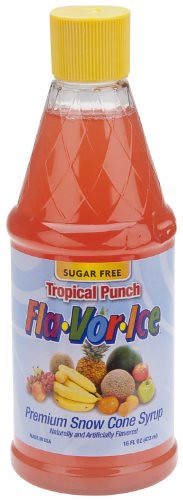In this detailed image, we see the design for a vertical bottle of Flavor Ice, a premium snow cone syrup. The bottle features a yellow cap adorned with vertical lines. Below the cap, the top portion of the bottle is cone-shaped and filled with an orangish-red liquid that extends down to the label. 

The label, occupying the bottom section of the bottle, is vivid and eye-catching. At the top of the label, "Sugar-Free" is prominently displayed in black text on a yellow background. The main body of the label is a mix of blue and white, with the product name "Flavor Ice" spelled out in colorful, vibrant letters. Below the name, there is an assortment of various fruits depicted in different shapes, sizes, and colors, highlighting the product’s fruity essence.

Further down, the label reads "Premium Snow Cone Syrup" in blue text, followed by the description "Naturally and Artificially Flavored." The quantity "16FL-OZ" and the statement "Made in the USA" are also printed on the label for additional information. The bottom section of the bottle is filled with the same orangish-red liquid, completing the attractive and flavorful design.